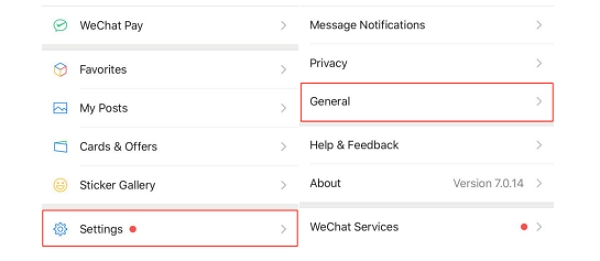This is a high-quality screen capture from a settings menu with a white background and black and gray text, divided into distinct categories separated by thin gray lines. 

At the top is the category "WeChat Pay," accompanied by a small green bubbly icon. Below it is "Favorites," with a blue, gold, and pink box icon. The next category, "My Posts," features a blue box with a white line icon. Following this is "Cards and Offers," represented by a blue card icon. "Sticker Gallery" comes next, symbolized by a gold emoji face. "Settings" is marked by a blue cogwheel icon and highlighted with a red dot and a red box around it.

On the right side, there are additional categories: "Message Notifications," "Privacy," and "General," with "General" also highlighted by a red box. Below these are "Help & Feedback" and "About," with the version number "7.0.14" noted next to it. At the bottom, there's a category labeled "WeChat Services," marked with a red dot and a gray arrow.

Each of these categories has a small gray arrow to the right, indicating they can be clicked. The image is in excellent quality without any pixelation or blurring, making all text and icons easily readable. There are no other notable objects present in the image.